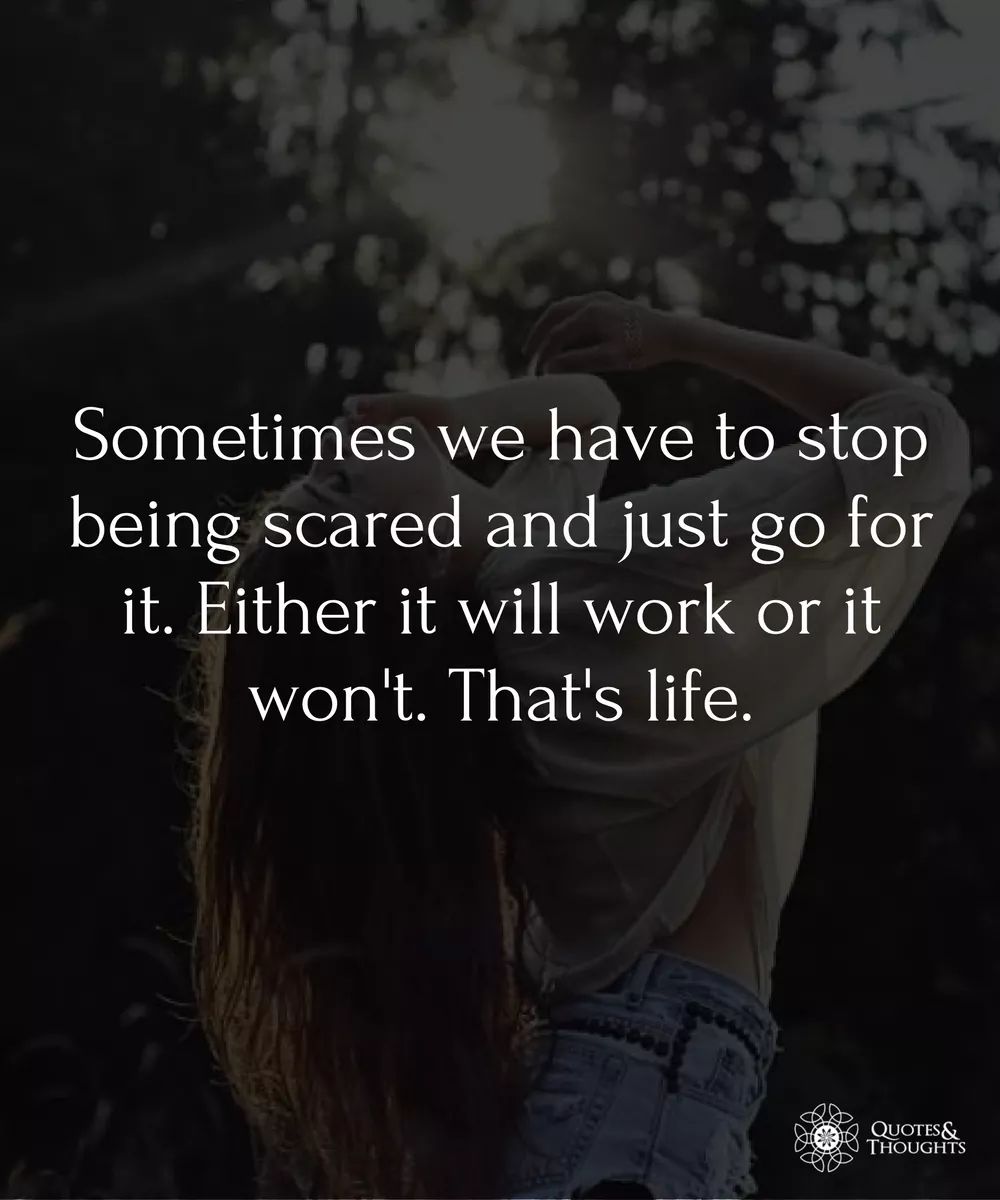The image is a rectangular poster, approximately six inches tall and five inches wide, with a very dark, tinted black background. The focal point is a young girl of Caucasian descent, standing against what appears to be a tree line with sunlight filtering through the trees at the top. The girl is wearing bleached blue jeans and a white sheer shirt. Her long brown hair, which hangs down below her waist, is dramatically tilted back. One of her arms is raised, with her elbow up in the air and her hand close to her face, appearing to dangle something into her open mouth.

Overlaid on this background, bold white text reads: "Sometimes we have to stop being scared and just go for it. Either it will work out or it won't. That's life." In the lower right-hand corner, there is a white circular symbol surrounded by three clover-like shapes. To the right of this symbol, the words "quotes & thoughts" are printed, with an ampersand underneath.